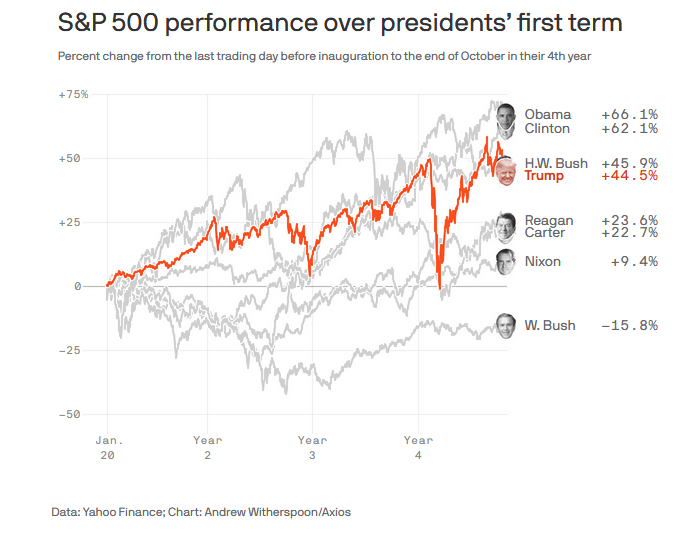The image features a detailed line graph titled "S&P 500 Performance Over President's First Term." The graph illustrates the percent change in the S&P 500 from the last trading day before each president’s inauguration to the end of October in their fourth year. 

On the vertical axis, the graph ranges from -50% to +75%. Horizontally, it starts from January 20 and marks through Year 2, Year 3, and Year 4. The graph includes data for Presidents Obama, Clinton, George H.W. Bush, Trump, Reagan, Carter, Nixon, and George W. Bush, each represented through a line or bar beside their names and percentage performances.

Obama leads with a performance of +66.1%, followed closely by Clinton at +62.1%. George H.W. Bush and Trump are at +45.9% and +44.5% respectively, with Trump’s data highlighted in red. Reagan follows with +23.6%, then Carter at +22.7%, Nixon at +9.4%, and George W. Bush showing a negative performance at -15.8%.

Each president's performance is color-coded in gray except for Trump, who is highlighted in red. The graph includes a note in the lower left corner citing "Data: Yahoo Finance, Chart: Andrew Witherspoon, Axios." The background is white, and the header text is prominently displayed in bold black print, with additional details in lighter print beneath.